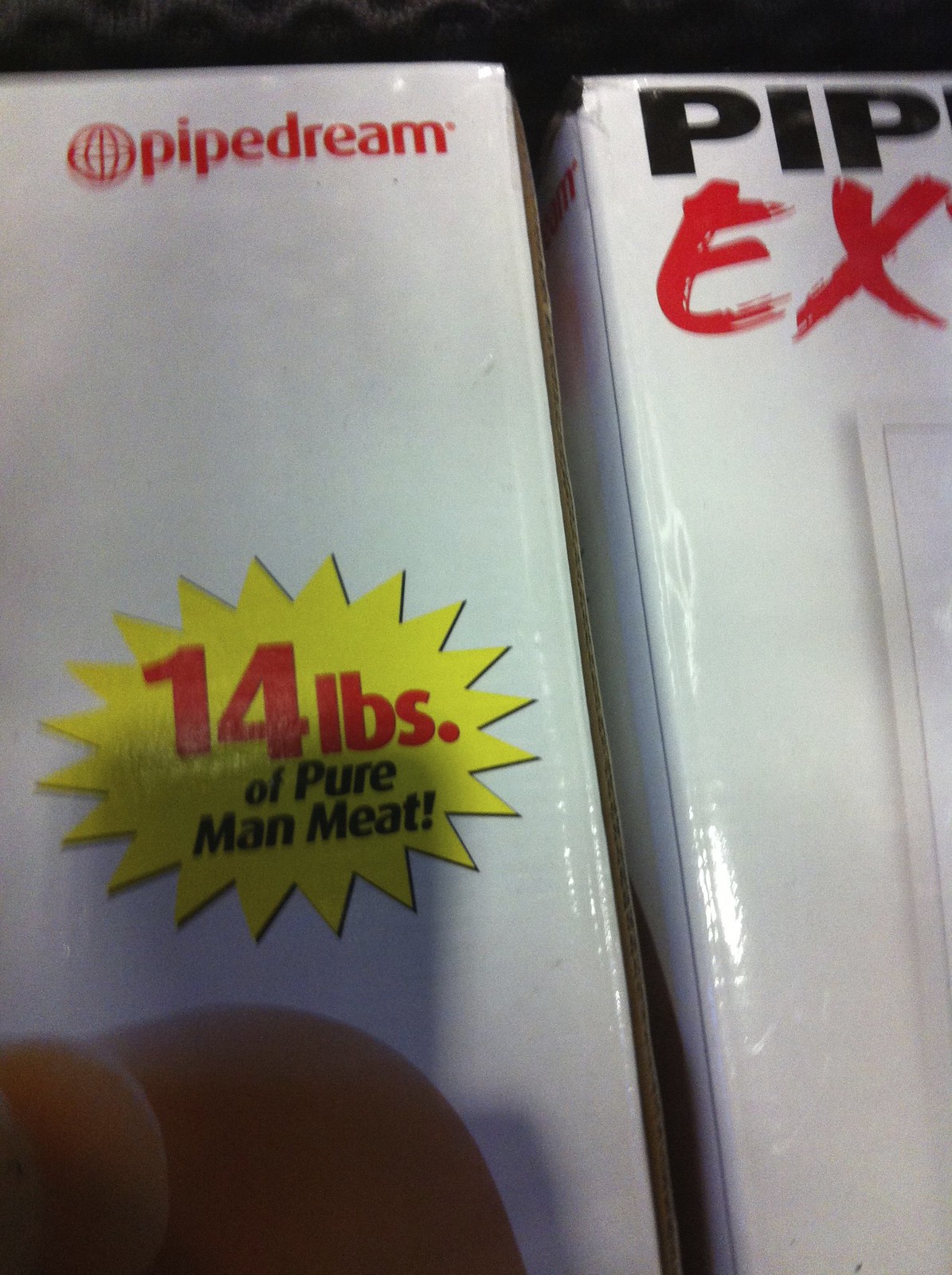In the image, there is a close-up of two packages wrapped in clear plastic. 

The package on the left features a white box displaying the brand "Pipe Dream" in red text at the upper right-hand corner, accompanied by a red globe icon. Below this, there is a vivid yellow sunburst graphic within which the text "14 pounds" is inscribed in bold red letters, followed by the phrase "of pure man meat" in black. Partially visible beneath this sunburst is a nude-colored item, though its exact identity is obscured by shadows.

The package on the right is also a white box. It prominently displays the word "PIPE" in large capital black letters, although only the letters "P.I.P." are fully visible. Beneath that, in stylized red brushstroke text, is the beginning of a word, starting with "X." The remainder of the package remains white, with any additional details or images obscured from view.